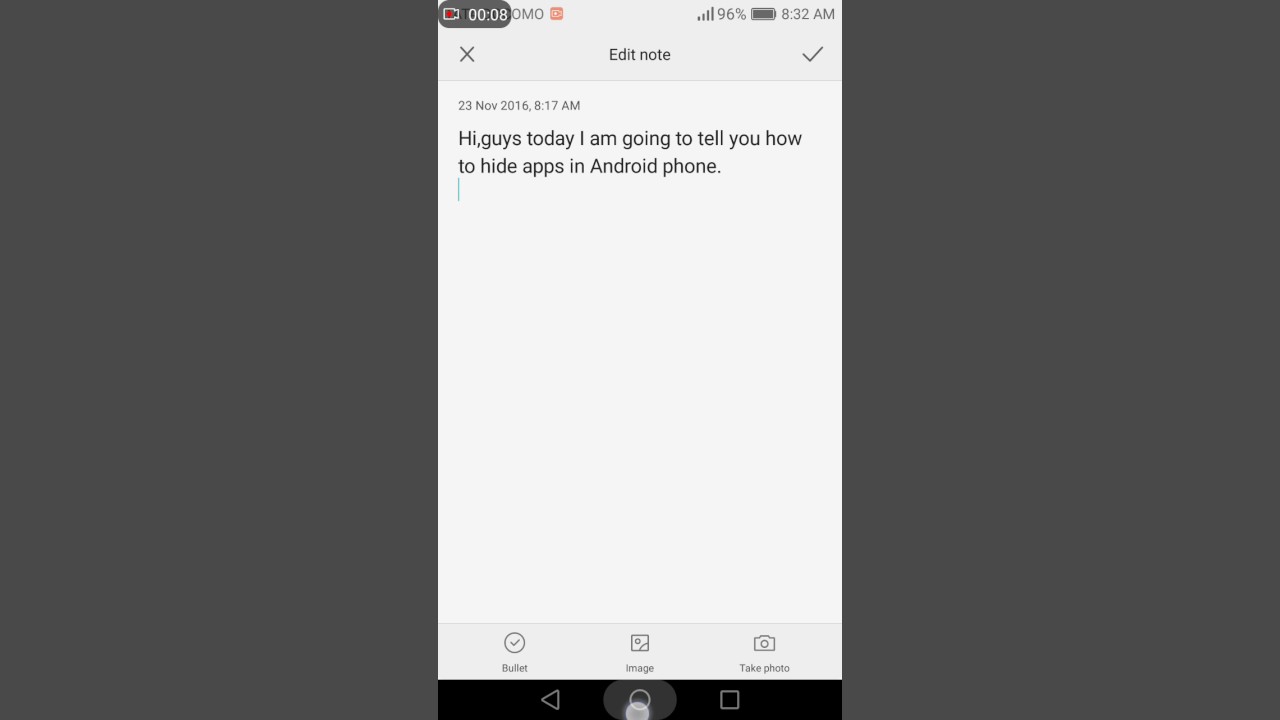Here is a refined and detailed caption for the described screenshot:

---

The screenshot displays a mobile phone interface. The screen is divided into three vertical sections: the leftmost third features a dark gray background, as does the rightmost third, leaving the central area to show the phone’s display. 

In the top right corner of the phone display, a small section of text is visible. Partially obscured by the gray background, the word "OMO" appears, overlapped by a gray oblong shape marked with "0.00008" in black text and a small red element inside it. 

Moving further right, the notification bar indicates the current time as 8:32 a.m. Next to it, the battery icon shows a nearly full charge at 96%, and there is an indicator with the number 4 representing internet connectivity. 

Below this top section, on the left side, there is a gray border encompassing an "x" icon in its center labeled as “Edit Note.” To its right is a checkmark within the same gray border. Beneath this area, against a white background, is a small line of black text reading "23 November 2016, 6:17 a.m."

The main body text, written in slightly larger black font, reads: “Hi, guys today I’m going to tell you how to hide apps in your Android phone.” Below this line is a visible cursor.

Extending to about two inches from the bottom of the screen, there is a thin gray border. On the right side within this border, there is a small black circle with a checkmark and the label "Bullet" beneath it. In the center of this lower section, an icon labeled "Image" is shown with an adjacent image placeholder. To the right, there is a camera icon labeled “Take Photo.”

Further down and to the right, various icons appear: a gray circle, a gray square, and a sideways gray triangle pointing left.